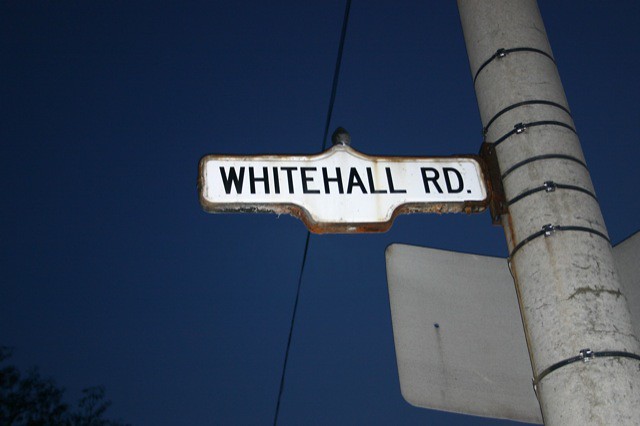In this landscape-oriented image, the primary focus is a street post featuring a road sign that prominently displays "Whitehall Road" in bold, clear black letters against a bright white background. Despite some rust patches visible on the sign, the text remains unfaded and easily legible. Below the "Whitehall Road" sign, an additional sign is attached, but it's oriented in the opposite direction. The post, which rises along the right-hand side of the image, is a light gray color, matching the tone of the signs. Stretching vertically from the top to the bottom of the image is a power line, likely extending from the pole featured to another one out of the frame. The background sky is a deep, dark blue, suggesting the image was taken around dusk. In the bottom corner, a few leaves are visible, hinting at the presence of a nearby tree. The photograph captures the scene from a low angle, possibly ground level, looking upwards, thereby highlighting the road sign as the central element of the composition.